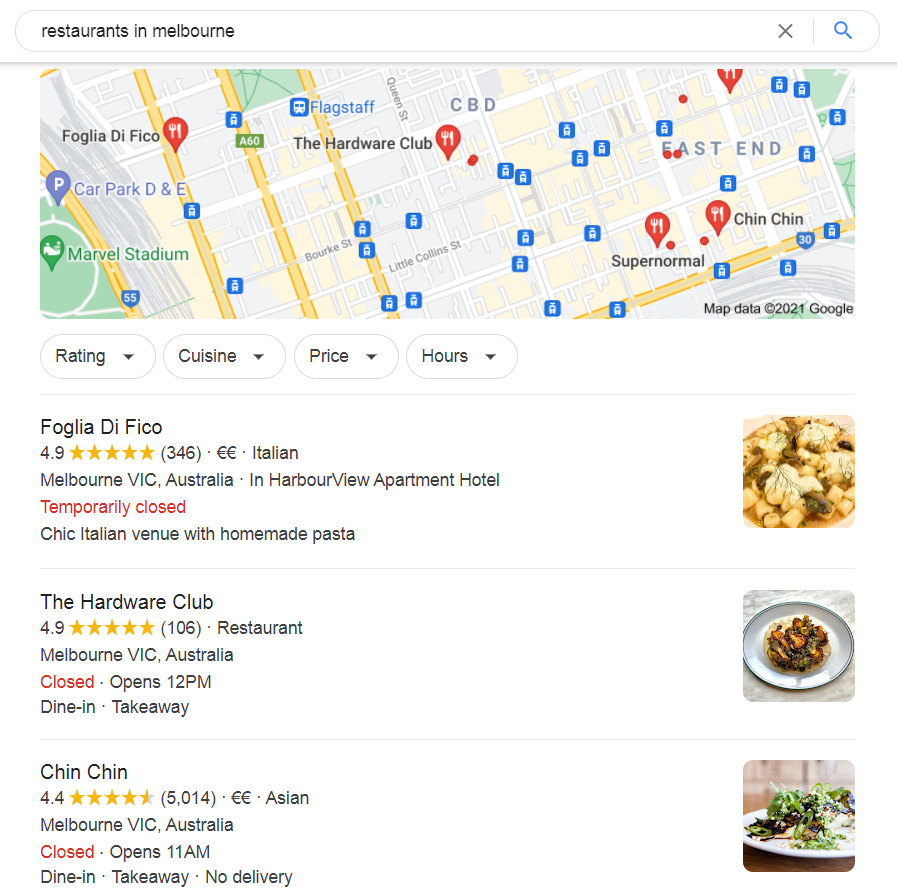This screenshot captures a Google search page for "restaurants in Melbourne" against a clean, white, and symmetrical background. The search bar is prominently positioned at the top, forming a long horizontal rectangle with a blue magnifying glass icon to its right and a white 'X' for canceling the search to its left. In the black font within the search bar, the query "restaurants in Melbourne" is clearly displayed.

Below the search bar, a map of Melbourne is featured, dotted with red balloon icons representing restaurants, each marked with a knife and fork symbol. Numerous small blue icons indicate transportation options like trains or buses. The map also highlights Marvel Stadium with a green hotel icon.

To the left of the map, a vertical list of restaurants is shown. The first entry is "Foglia Di Fico", noted as temporarily closed with an impressive 4.9-star rating and a cost symbol of two Euros, signifying a moderately expensive option. A picture of the food from this restaurant is displayed to its right.

Below it, the "Hardware Club" is listed, also closed, with a 4.9-star rating. This restaurant offers dine-in and take-away options, as indicated by its description. A small plate of food is pictured alongside its listing.

Further down is "Chin Chin", boasting a 4.4-star rating from 5,014 reviews. This Asian restaurant, which has a moderate cost indicated by two Euros, is closed currently but will reopen at 11 a.m. Located in Brick, Melbourne, Australia, it offers dine-in and take-away services but does not provide delivery.